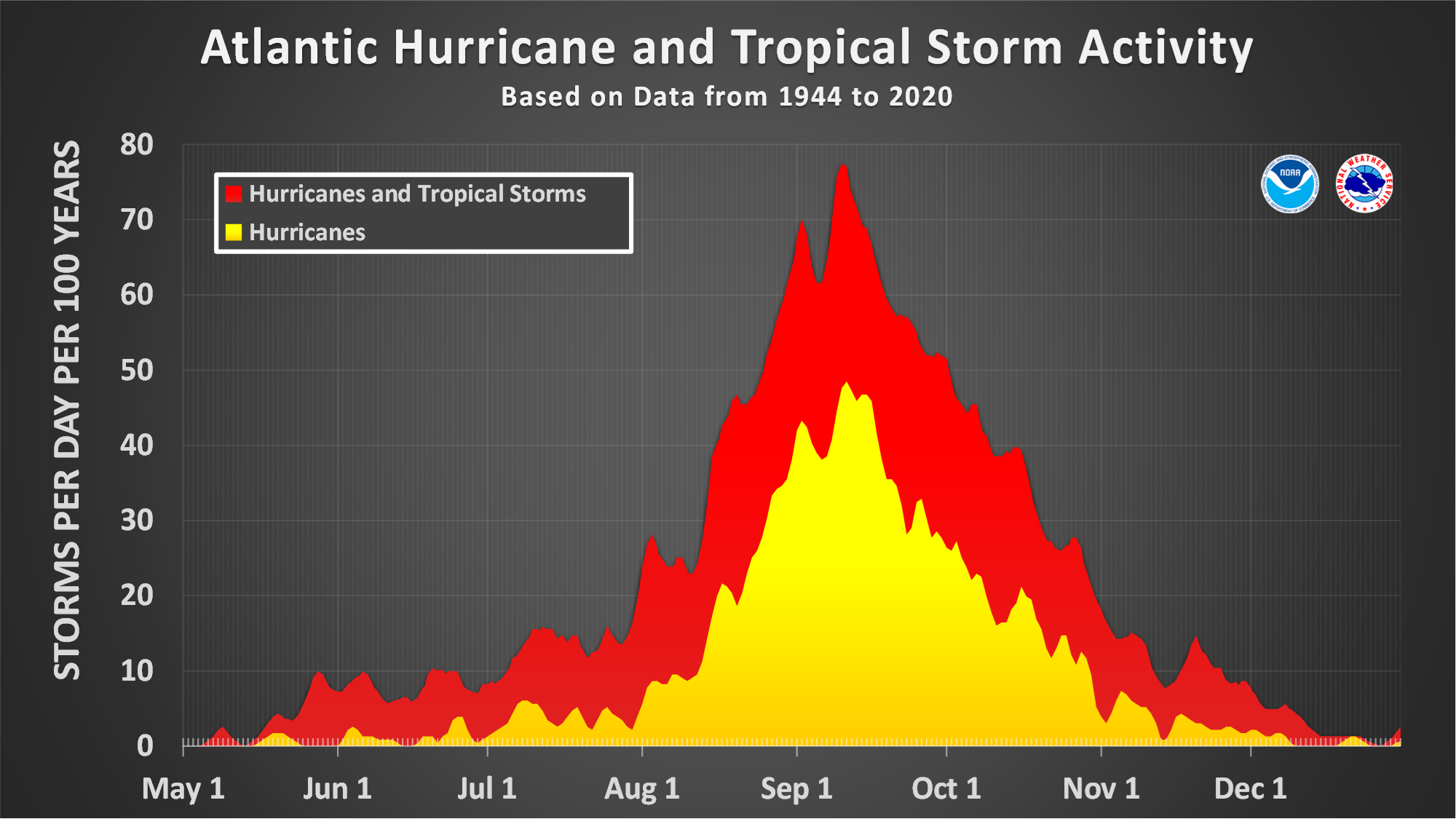This detailed diagram, resembling a textured filled graph on a dark gray background with a light gradient center, illustrates "Atlantic Hurricane and Tropical Storm Activity." The title is prominently featured in white text at the top, with a subtitle underneath in smaller letters stating, "based on data from 1944 to 2020." The y-axis on the left side is labeled "storms per day per 100 years," ranging from 0 to 80 in increments of tens. Horizontally across the x-axis, time is marked from May 1st to December 1st, highlighting the months.

The graph uses two colors: red represents both hurricanes and tropical storms, while yellow signifies only hurricanes. The overlapping textures of these two categories form a distinct pattern showcasing peak storm activity. The red hurricane and tropical storm activity reaches up to about 70 per day per 100 years at its peak, while the yellow hurricane-only data spikes to around 50 per day per 100 years. The peak period for both categories spans from early September to early October, forming a bell curve with significantly lower activity at the beginning and end of the period.

In the upper right corner of the graph, two small circular logos appear, likely representing governmental or meteorological organizations. One of these logos may be from FEMA, while the other features blue in the center with red lettering around the outside.